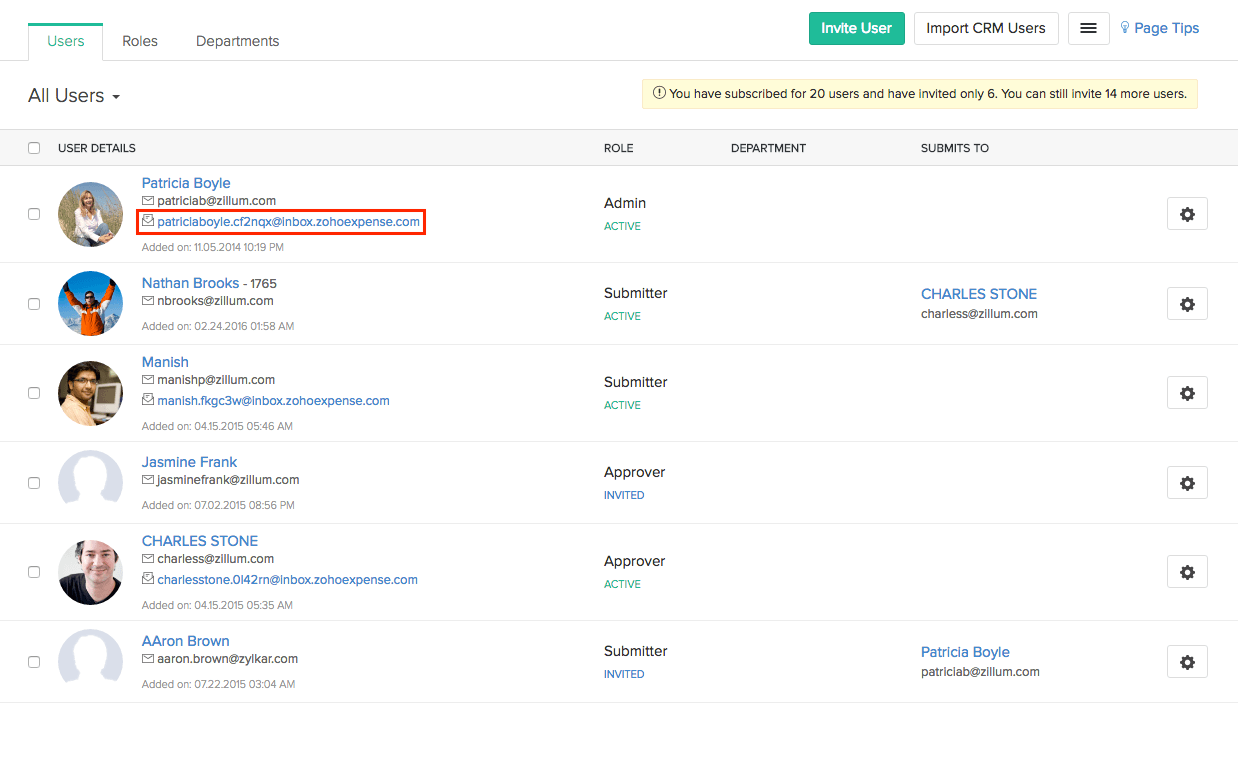The interface displays three primary tabs at the top: "Users," "Roles," and "Departments." The "Users" tab is currently selected, highlighted in green. Below these tabs, there is a green button labeled "Invite User" and a white button labeled "Import CRM Users." A hamburger menu button is also present, along with a blue hyperlink labeled "Page Tips."

A drop-down menu titled "All Users" allows for filtering options. The main content area is organized into four columns, which from left to right are labeled: "User Detail," "Role," "Department," and "Submits To."

Three user entries are listed in the table:
1. Patricia Boyle, email: patriciab@xilm.com, with an extended string of information trailing her email, was added on 11-05-2014 at 10:19 PM.
2. Nathan Brooks, ID: 1765, email: nbrooks@xilm.com, was added on 02-24-2016 at 01:58 AM.
3. Manish, email: manishp@xilm.com.

Each entry provides detailed information about the user, including their role, department, and submission details (not specified in the provided text).